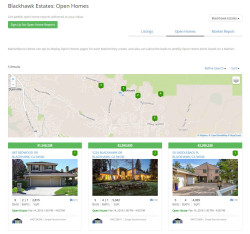This image depicts a small, somewhat hard-to-read map focused on Black Hawk Estates, highlighting homes available for sale in that area. The central section of the image showcases a map with five prominent markers, though only three homes are listed below due to cropping. The homes appear to be in a suburban setting—one is confirmed to be a two-story building, while the details of the other two remain unclear. The color scheme predominantly features whites, complemented by green accents around the buttons and map markers. The background landscape of the map shows typical terrain with a distinct green area near the top, possibly indicating a forested region or a nearby mountain. The image provides a snapshot of the real estate listings within the Black Hawk Estates, yet lacks specific details such as prices, number of bedrooms, or exact location identifiers.